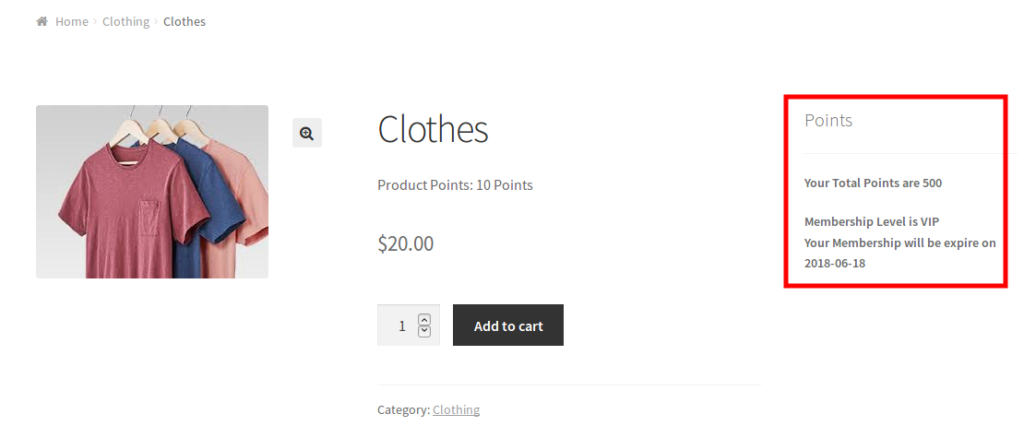Screenshot from an online clothing store interface:

The screenshot features a minimalistic layout with a white background. In the upper left corner, there's a grey house icon followed by navigation links: "Home" and "Clothing". Below, there is a grey-scale image showcasing three shirts on wooden coat hangers. The shirts are in three colors: reddish, bluish, and light tan.

To the right of the image, the text reads "Clothes" with a subtitle "Product" marked with 10 points, priced at $20. Below, there is a grey box with a number "1" and up/down arrows for selecting the quantity. Adjacent to this is a black "Add to Cart" button in white text.

On the right-hand side, a box outlined in red contains membership details. The text starts with "Points" in light grey and follows with more details in a darker grey or light black font: "Your point totals are 500. Membership level is VIP. Your membership will expire on 2018-06-18."